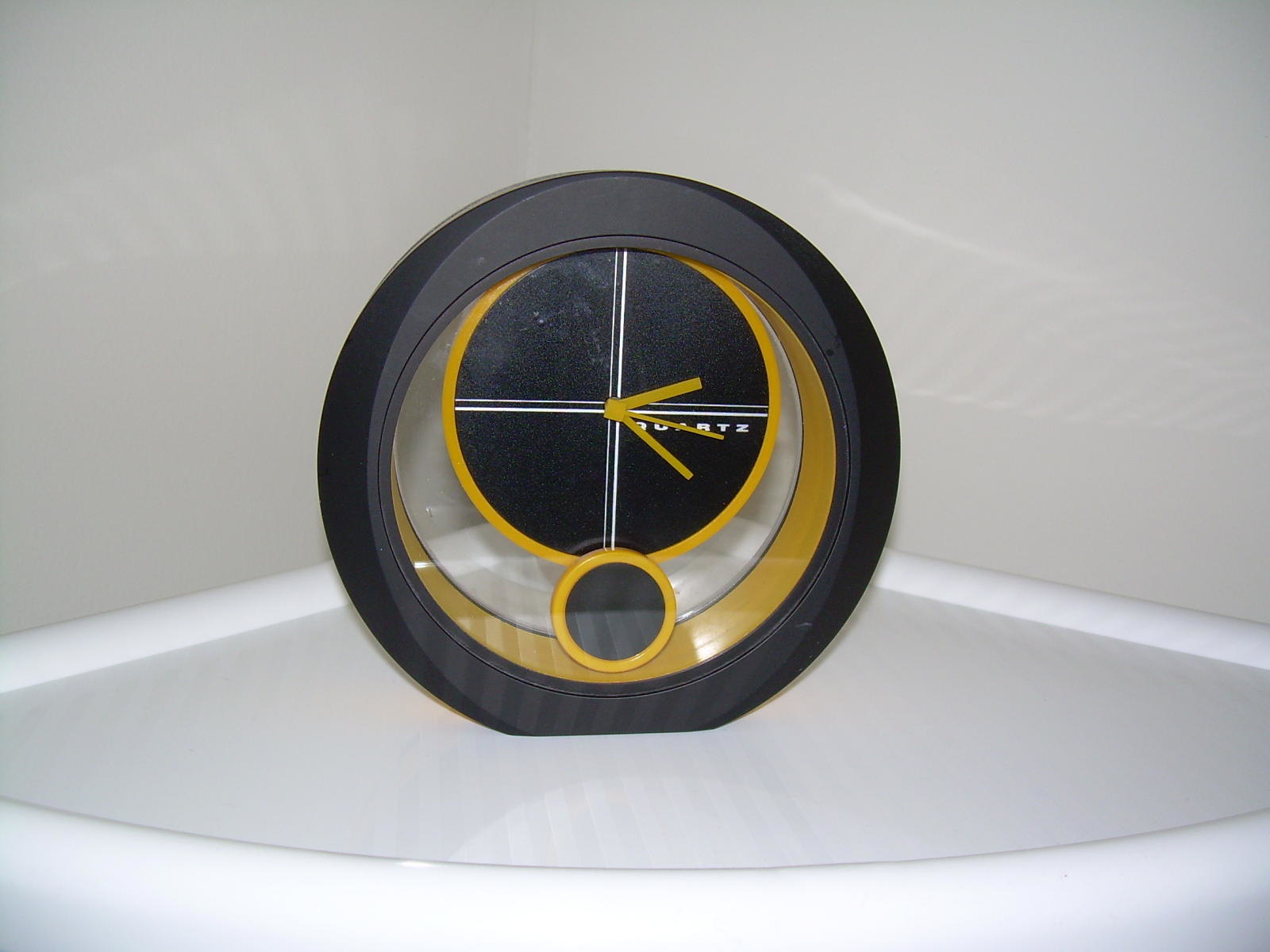In the image, a corner shelf is integrated into the light gray walls of a room, creating the impression of a seamless, built-in structure. The shelf is white and has a rounded front edge, perfectly nestled into the corner. Dominating the shelf is a distinctive round clock. The outer casing of the clock is black, contrasting with the clear glass or plexiglass front that protects the face. 

Inside the clock, the deep cylindrical cavity is lined with a vibrant yellow inner ring, and the back of the clock is white. The clock face itself is quite minimalistic, featuring no numbers, only intersecting white lines dividing it into quadrants from 12 to 6 and 9 to 3. The black face of the clock hosts yellow hour, minute, and second hands, with "Quartz" inscribed in white letters towards the lower right section. Directly beneath the main face is a smaller yellow circle with a black dot inside, the function of which is unclear; it might be an alarm indicator or a speaker. The clock's face is glossy, reflecting the surrounding light and adding to its modern, sporty aesthetic. Adding to the simplicity and focus, the photo captures a predominantly white and gray palette, drawing your attention to the striking design of the clock against the understated background.